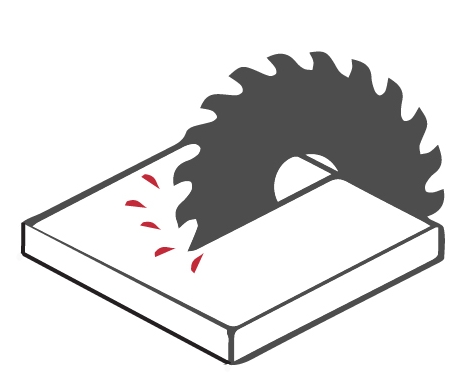On a stark white background, this warning infographic depicts a detailed, three-dimensional, dark gray square block being sliced by a dark gray circular saw blade. The image emphasizes the danger by showing the blade cutting halfway through the block at an angle, with the blade's teeth curving slightly downward. On the upper right surface of the block, near the point where the saw blade cuts through, small red drops signify blood, accentuating the potential hazard.Outlined in black for clarity, the simplistic yet striking black, white, and red color scheme serves to draw attention to the risk associated with improper use of a table saw.